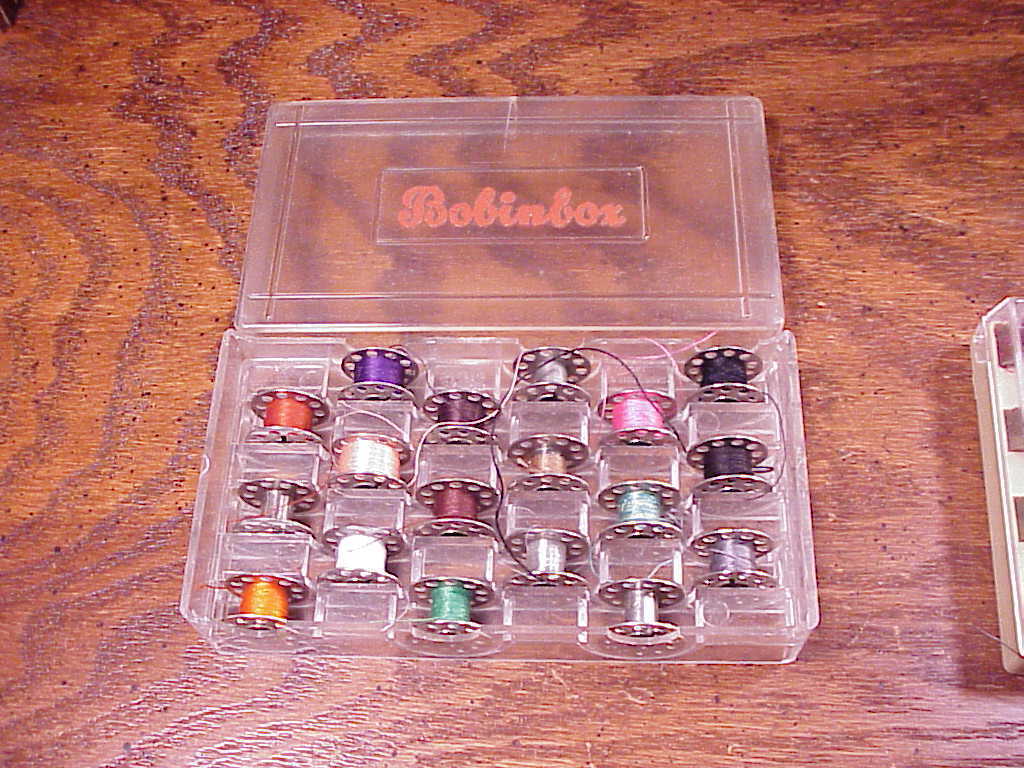The image features a translucent plastic box labeled "bobbin box" in orange text, placed centrally on a wooden surface, likely a table or counter in an indoor setting such as an arts and crafts room. Inside the box are 18 bobbins, four of which are empty, wound with thread in various colors including black, white, off-white, different shades of brown, red, orange, silver, purple, pink, green, beige, tan, and multiple shades of orange. The spools are neatly arranged and predominantly silver in appearance. An indistinct translucent plastic object is partially visible off to the right side of the frame.